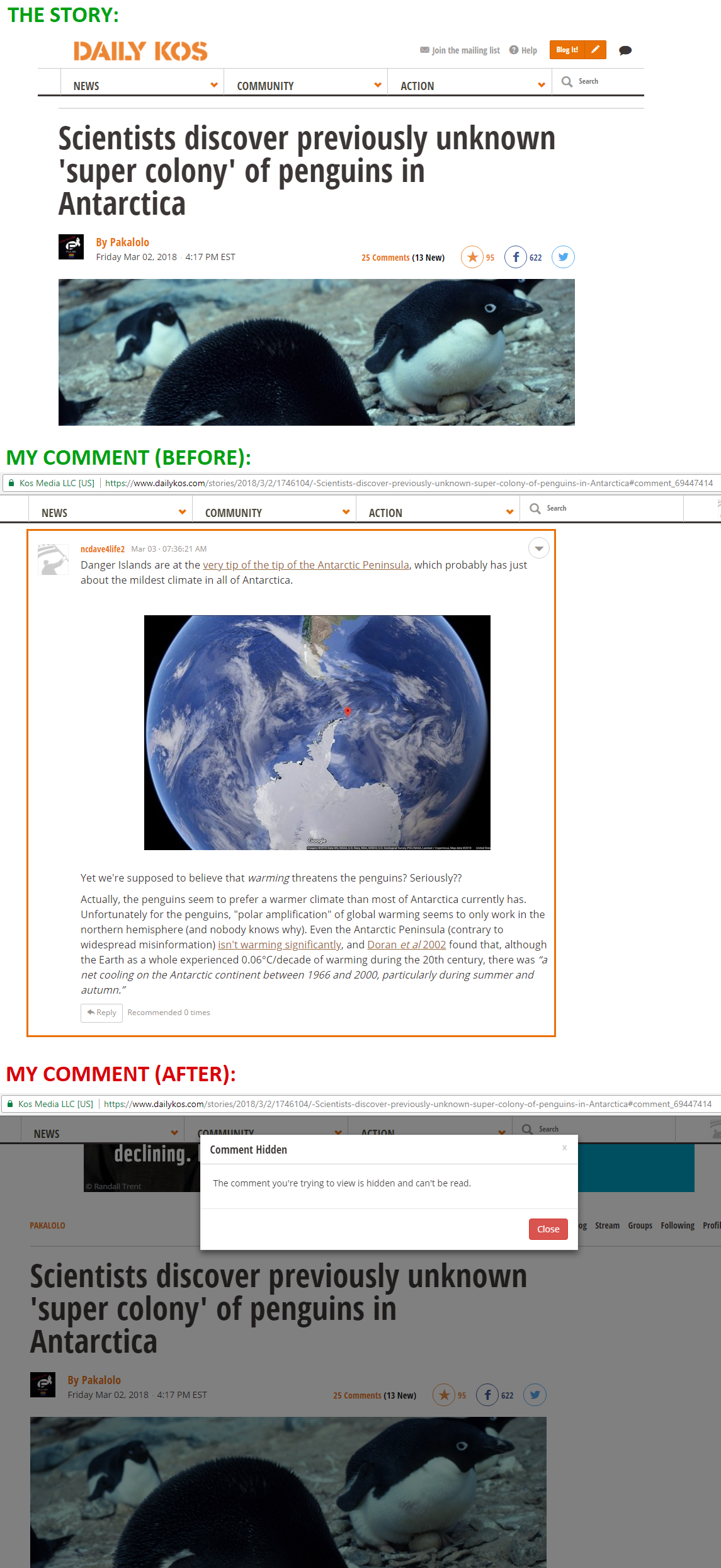A smartphone screen displays a news article on the website Daily Calls, a platform known for its NEWS, COMMUNITY, and ACTION sections. The top of the screen prominently features the site's green-colored header with the title "THE STORY" in all caps. Below this header, the navigation options NEWS, COMMUNITY, ACTION, and a SEARCH BAR are visible.

The main headline of the article, written in bold black letters and enclosed in quotation marks, reads: "SCIENTISTS DISCOVER PREVIOUSLY UNKNOWN SUPERCOLONY OF PENGUINS IN ANTARCTICA." Above the headline is the byline, while just below, there is a high-resolution, close-up image of penguins standing on an expanse of ice.

Further down, a green section labeled "MY COMMENT BEFORE" in parentheses appears, although its content is partially obscured and unreadable. Adjacent to this is a small world map highlighting Antarctica with a tiny red dot labeled "DANGER ISLANDS," though the text is too small to discern clearly.

Comments are featured in the article, with a section marked "MY COMMENT AFTER" in red, indicating user interaction. There is also a red button that users can press to hide or display this comment section.